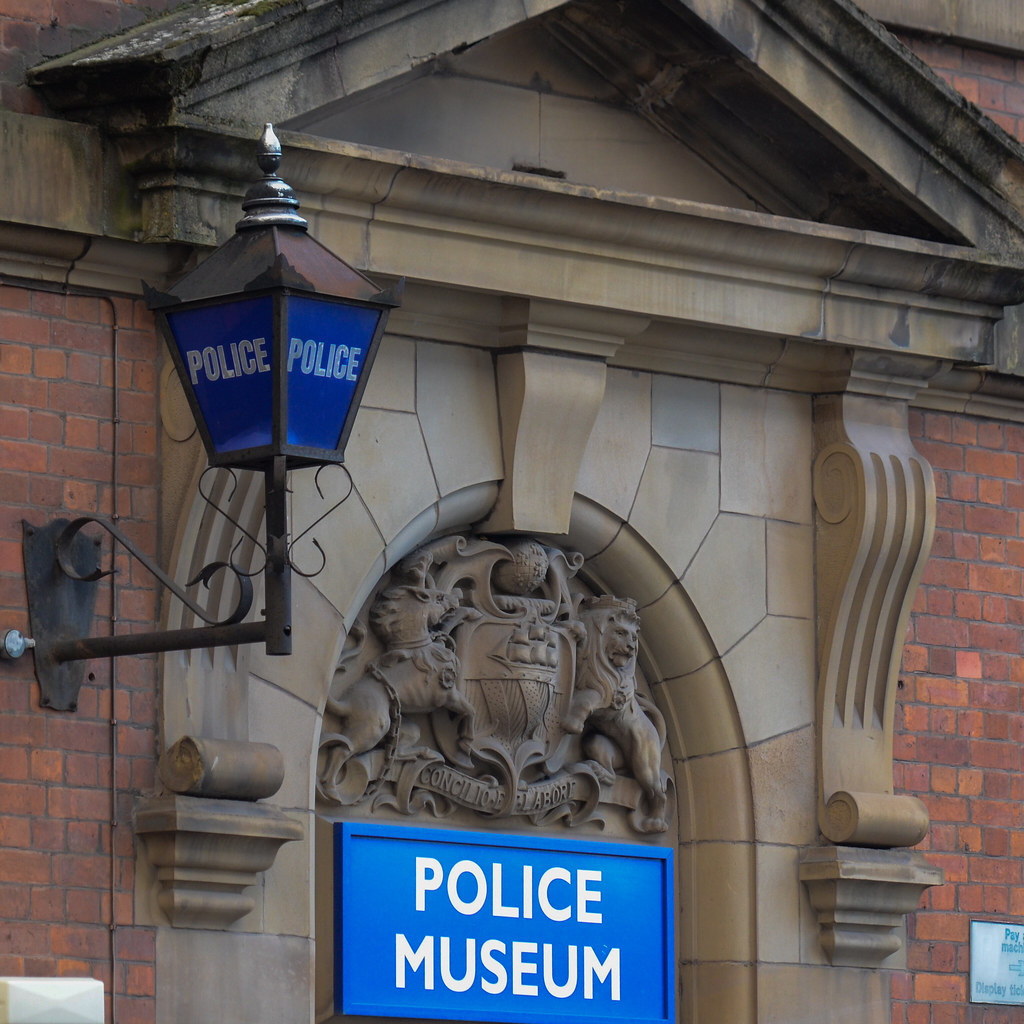This image captures the front facade of a Police Museum building. The central feature is a prominent stone archway encased in light gray stone, which is very well maintained. Flanking the archway are red brick walls. Above the archway, there is an intricate stone sculpture featuring a lion on the right, a horse—or possibly a unicorn—on the left, and both appear to be surrounding a shield. Beneath this sculpture, a blue plaque with white text clearly reads "Police Museum."

To the left of the archway, an old-fashioned black metal lamppost with blue panes bearing the word "POLICE" in white is mounted on the brick wall. Just below it, on the extreme bottom right of the image, there is a partially visible white plaque with teal-colored writing, with the words "pay" and "M-A-C-H" discernible. The upper portion of the image hints at a triangular pediment that comes up from the left and right sides toward the center but is cut off at the top of the photograph. The stone and brick elements combine to create a structured and historic appearance, emphasized by the ornate stonework and classic lamppost.